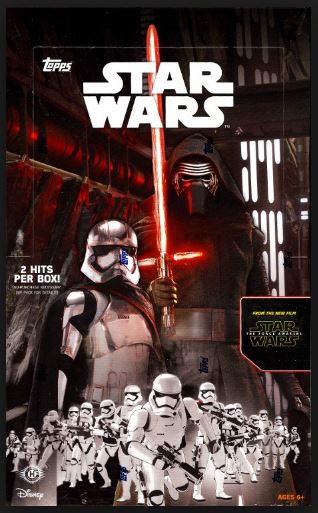This promotional graphic for the Star Wars franchise appears to be the packaging for a box of trading cards. Dominating the lower portion of the image are approximately 20 Stormtroopers arranged in a triangle formation, advancing towards the viewer with guns in hand. Centered at the top is the iconic white Star Wars logo, with another white logo for TOPS situated in the upper left corner. In the middle of the image, two prominent characters are featured: Kylo Ren, dressed in a black hooded outfit with a menacing mask and wielding a red cross-shaped lightsaber, and Captain Phasma, clad in her distinctive chrome and metallic armor with a white helmet and cape. Text on the left side of the image declares "two hits per box," hinting at some special feature of the trading cards. The recognizable Disney logo is displayed in the lower left corner, while the lower right corner has an orange text indicating "ages six plus." This detailed and vibrant graphic showcases a dynamic visual appeal, aiming to captivate Star Wars fans and collectors alike.